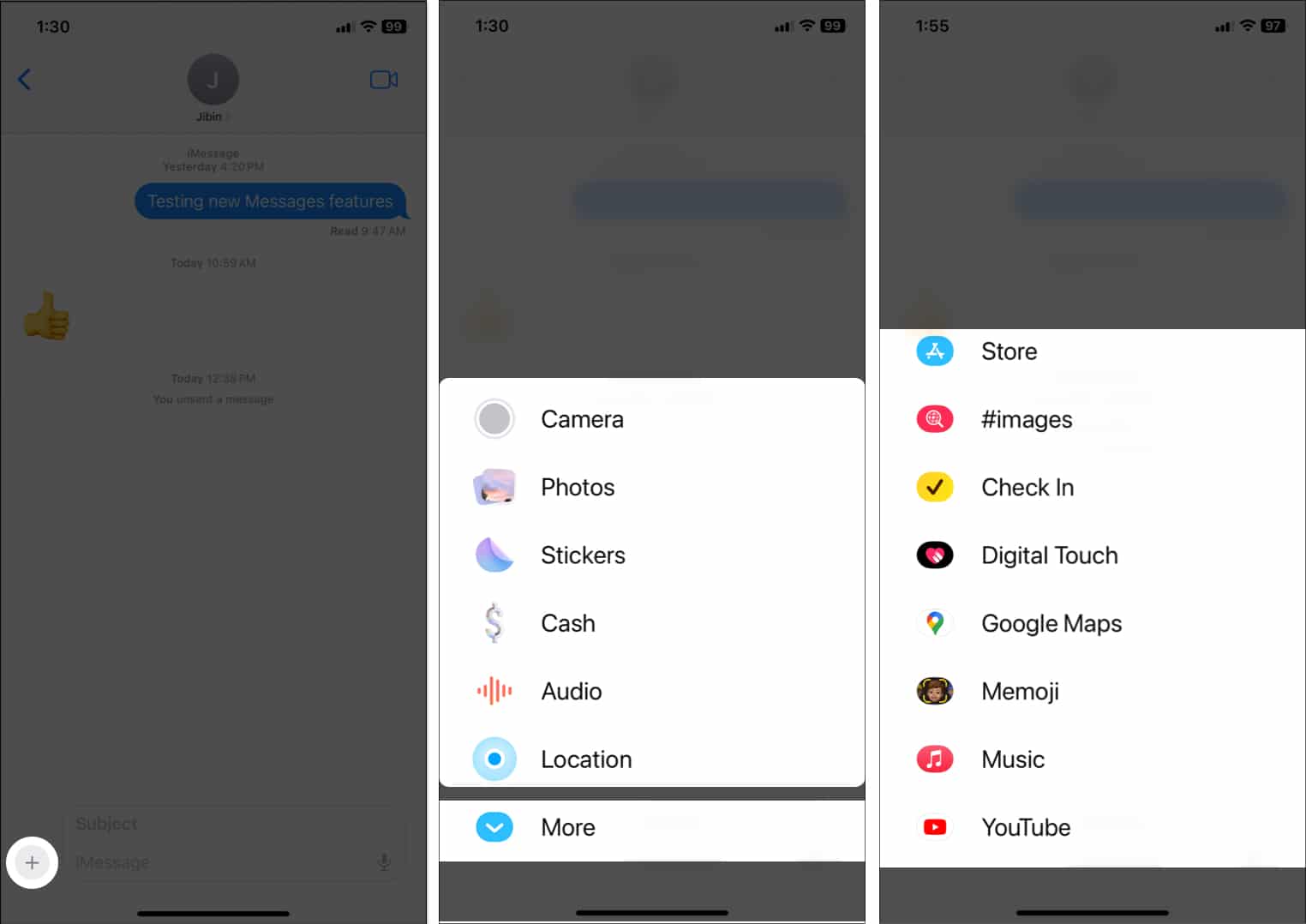This is a horizontally oriented rectangular image, showing three distinct screenshots from a cell phone, most likely an iPhone, arranged in a row. Each screenshot appears to be part of the same text messaging application.

In the first screenshot on the left, we see a primarily grayed-out screen, save for a small white circle with a plus sign located in the bottom left corner. Despite the grayed-out backdrop, the display faintly shows the time as 1:30 at the top left, along with the cell phone signal and Wi-Fi strength indicators on the top right. Within this muted text conversation, a thumbs-up emoji is visible, though the text itself is unreadable and the recipient's name is not shown.

Moving to the center image, the content of the text message remains consistent, as indicated by the same time, signal strength, and Wi-Fi indicators. Here, a white pop-up window dominates the foreground, presenting several selectable options: Camera, Photos, Stickers, Cache, Audio, Location, and More. Each of these options is associated with a corresponding icon, standing out against the persistent grayness of the background.

The third screenshot on the right introduces a new pop-up window, which features a list of multiple items, although the specific details of these items are not provided. The rest of the screen remains grayed out, maintaining the continuity of the visual theme across all three images.